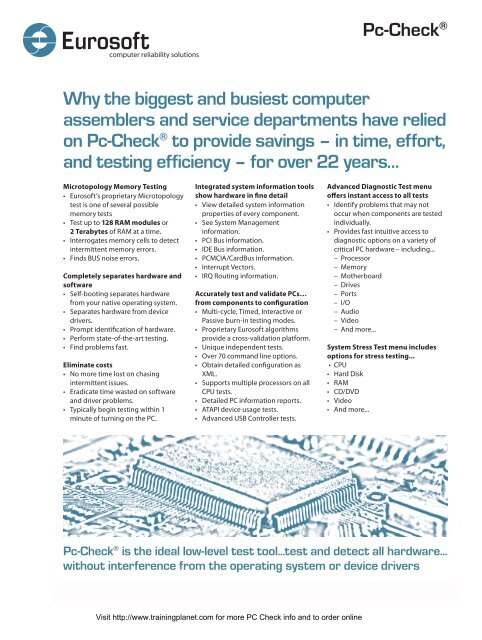This vertically-aligned informational page promotes Eurosoft's PC-Check, a software celebrated for over 22 years for its efficiency in testing and diagnostics. The top-left corner features "Eurosoft" in black letters accompanied by a blue and white circular logo, with "computer reliability solutions" inscribed underneath. Opposite, in the top-right, it boldly states "PC-Check." The title is prominently displayed in blue, left-aligned, reading: "Why the biggest and busiest computer assemblers and service departments have relied on PC-Check to provide savings in time, effort, and testing efficiency for over 22 years...". Below, three columns of detailed small black text enumerate the features and benefits of PC-Check, including micro topology memory testing and system stress test options. A blue and white rectangular illustration at the bottom, likely depicting various computer components, reinforces the theme. Beneath this, it asserts, "PC-Check is the ideal low-level test tool...test and detect all hardware...without interference from the operating system or device drivers." The fine black print at the page's foot concludes with the website: "www.eurosoft.com."